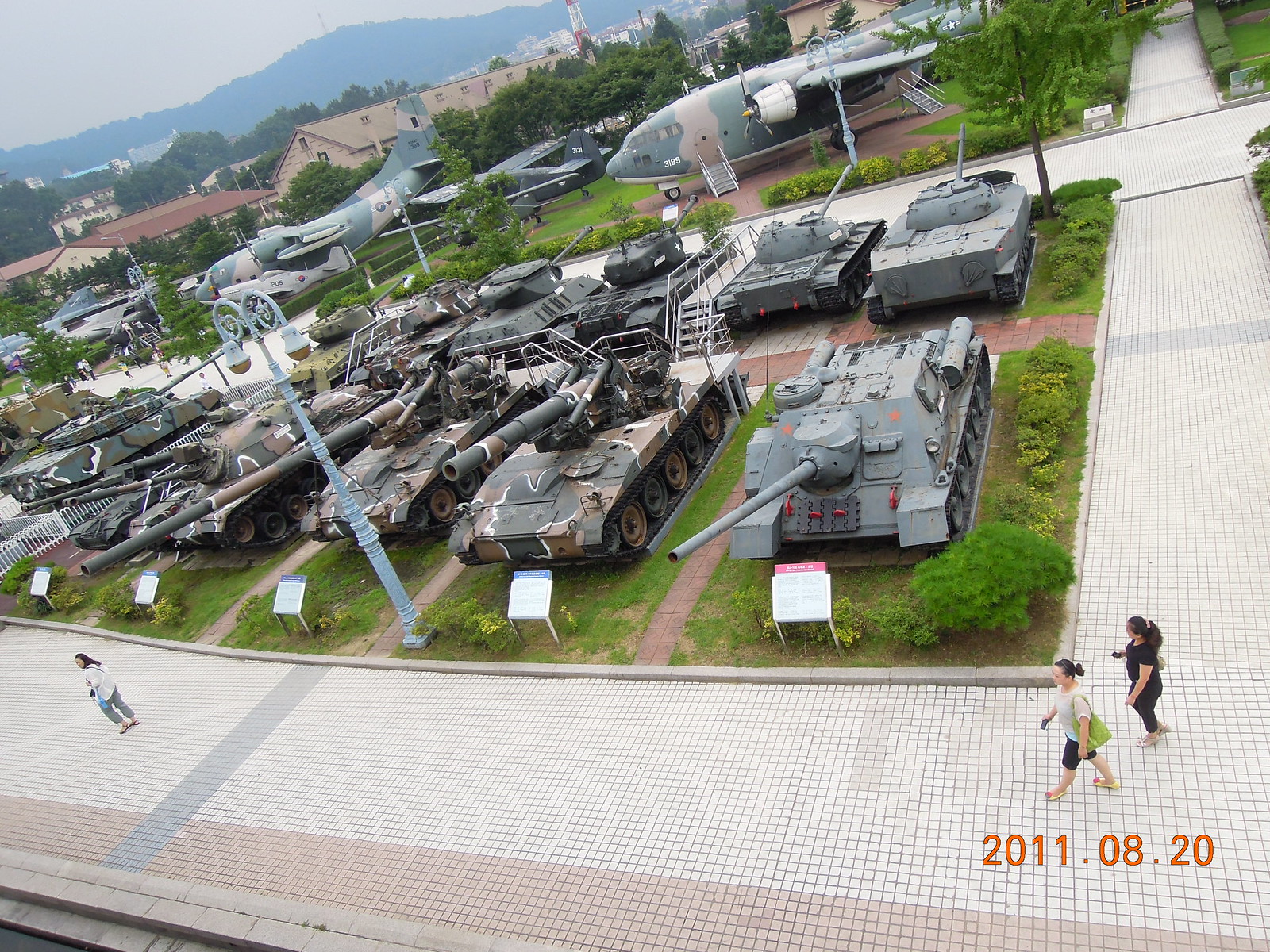This photograph, taken on August 20th, 2011, showcases an outdoor military vehicle display at what seems to be a military museum or open house event. The setting features a spacious layout with wide pathways made of white, brown, or gray tiles that could fit eight people across, forming organized, square-shaped display areas. Central to the photograph is a green grassy area containing about ten military tanks with long turrets, each positioned on individual grassy patches separated by brick pavers, with signs in front of each tank for informational purposes. Surrounding the tanks, you can see more display areas featuring various types of airplanes, including large bombers with camouflage paint. The scene is set against a backdrop of slightly overcast skies and distant mountains, creating a picturesque view. In the bottom right-hand corner of the photograph, there is a timestamp "2011.08.20." Additionally, three women are visible; two are walking from right to left along the tiled pathway on the bottom right side, and another is seen on the left side of the picture, also making her way to the left. The event appears to be open to families or the general public, given the casual presence of these visitors.